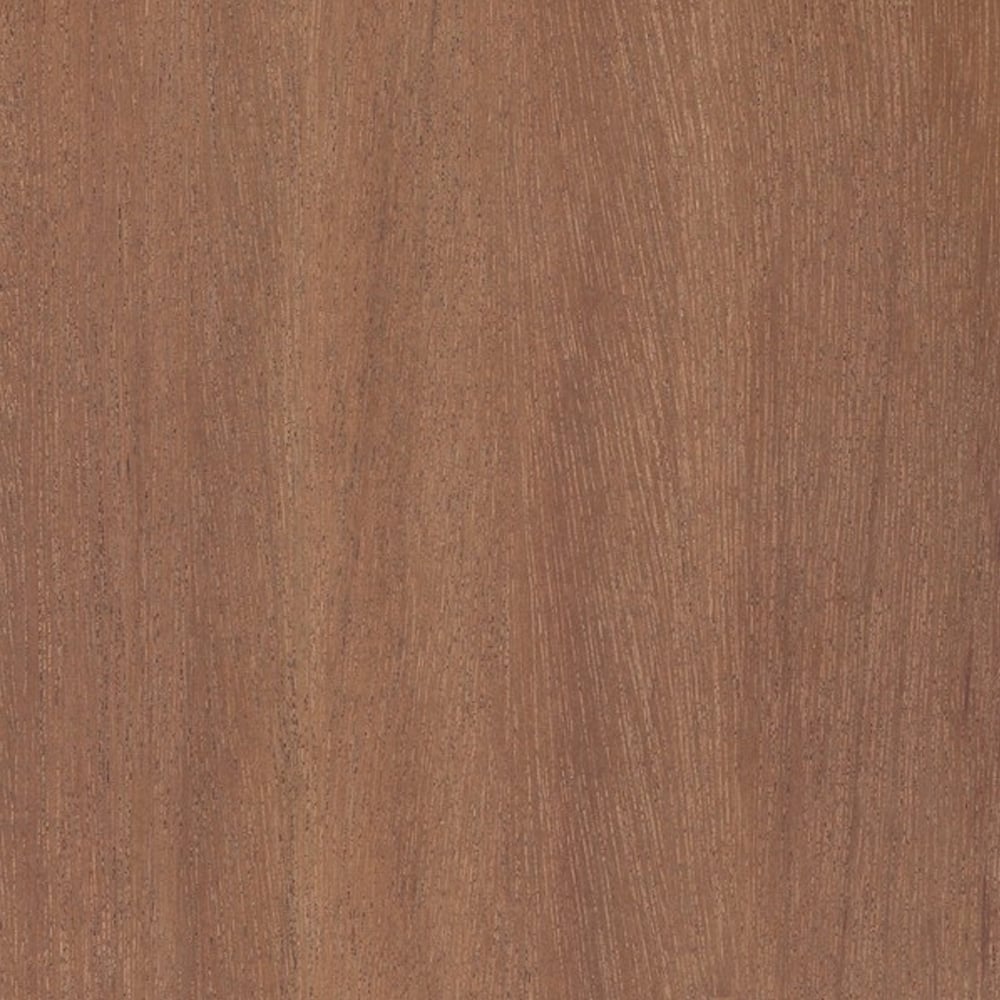The image portrays a detailed and close-up view of a medium brown, unfinished wooden surface. This square-shaped sample features distinct vertical wood grain patterns, with darker and lighter streaks that are particularly pronounced in the middle and towards the left. The absence of any objects or text around it, combined with its non-reflective, raw-coated finish, suggests it could be a highly zoomed-in shot of a wooden table or a similar wooden surface. The wood does not have a glossy, lacquered look, giving it a natural, untreated appearance. Its teddy bear brown shade makes it neither overly dark nor excessively light, striking a balance in the medium brown range.